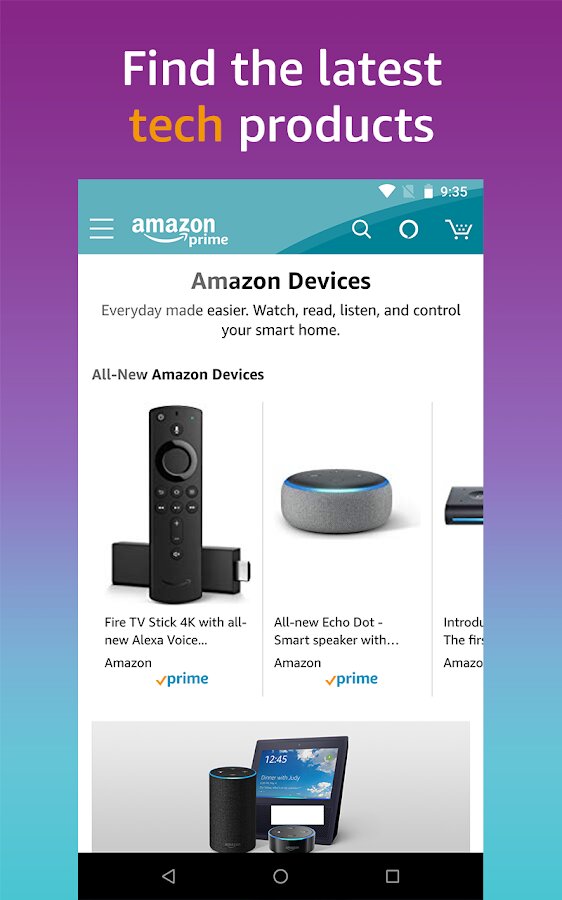The image prominently features a header text that reads "Find the Latest" on the first line and "Tech Products" on the second, located at the top center of the image. The background behind this text transitions from a purple gradient at the top to a light blue towards the bottom. Beneath the header, a screenshot of a smartphone extends down to the image's bottom center. This screenshot shows an Amazon webpage, specifically a section showcasing Amazon devices. 

In the screenshot, against a white block background under the Amazon logo, various tech products are displayed. The first product on the left is a Fire TV Stick 4K. Adjacent to it is the "All-New Echo Dot Smart Speaker." There is an additional item partially visible to the right, but it is cut off from the image. Below this display, there's an image featuring a circular smart speaker, resembling an Echo Dot, and a weather display screen with LED or LCD technology, indicative of a smart home device.